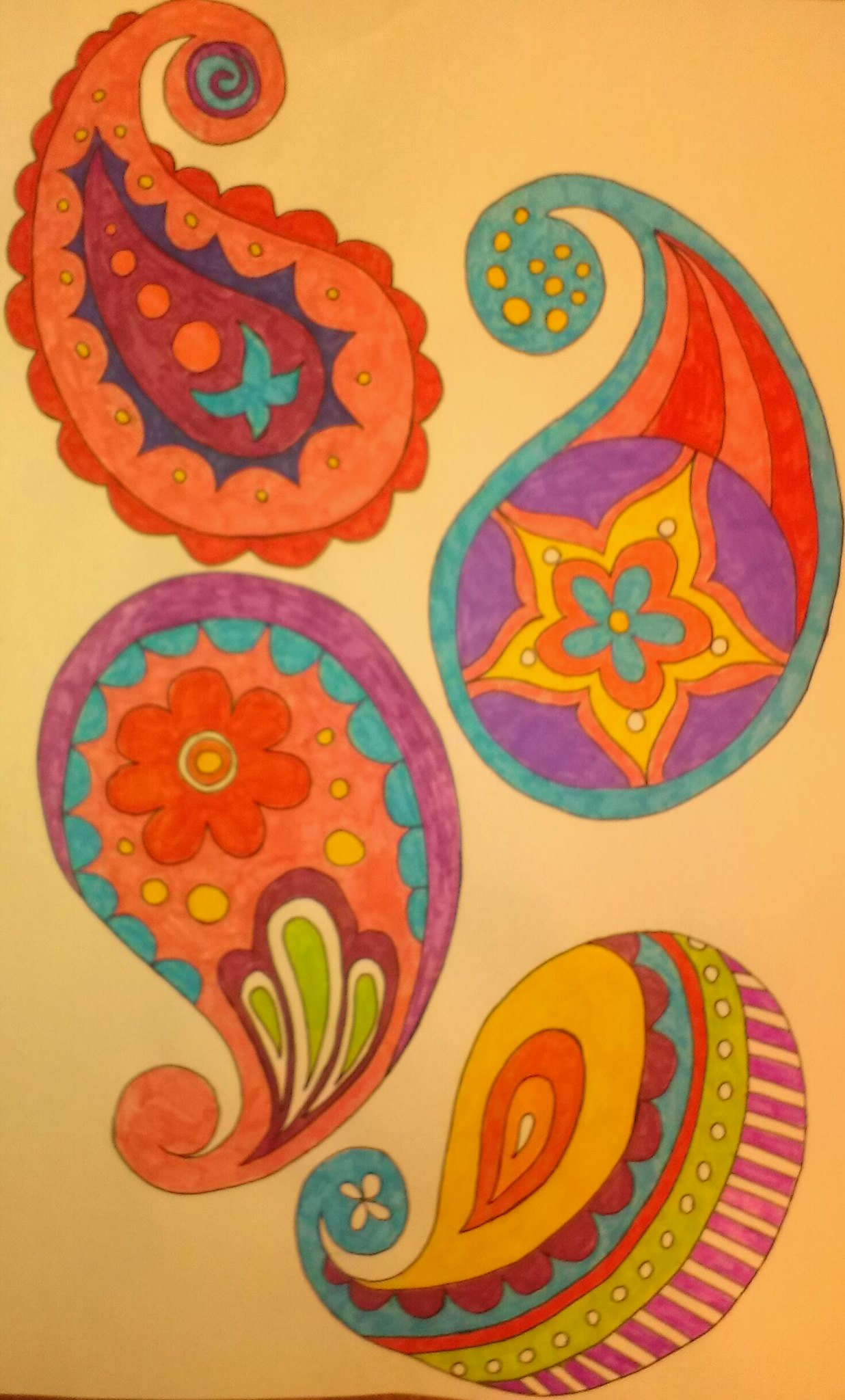This visually striking graphic art print features a vivid and dynamic composition set against a subtle mustard yellow background. At the forefront, four intricately designed paisley shapes, each resembling a teardrop with an elegant spiral at the narrow end, burst with color and pattern.

- In the upper left corner, a paisley shape dazzles with predominantly red and orange hues. It begins with a scalloped red outer edge, followed by a scalloped orange layer, a hint of purple, and then more red and orange accents. At its heart, a teal figure reminiscent of a butterfly adds an extra touch of whimsy.
  
- Moving down to the upper right, the paisley design starts with a teal exterior and radiates with orange and red stripes. It features a circular section at its base adorned with a yellow and orange star-like flower, highlighted by a purple border and a teal daisy at the center.
  
- In the lower right corner, the paisley shape exhibits a playful mix of pink and yellow stripes, punctuated by yellow dots on the same yellow background. It follows with an orange stripe, a teal stripe, a scalloped red segment, further layers of orange in varying shades, and finishes with a delicate yellow detail.
  
- Finally, the middle left paisley shape starts with a purple outer edge transitioning into teal. Layers of orange and darker orange follow, leading to an internal design featuring a lime green and yellow teardrop, bordered by a dark red outline.

The combination of these vibrant, diverse elements creates a lively and captivating artwork that is both colorful and visually pleasing.